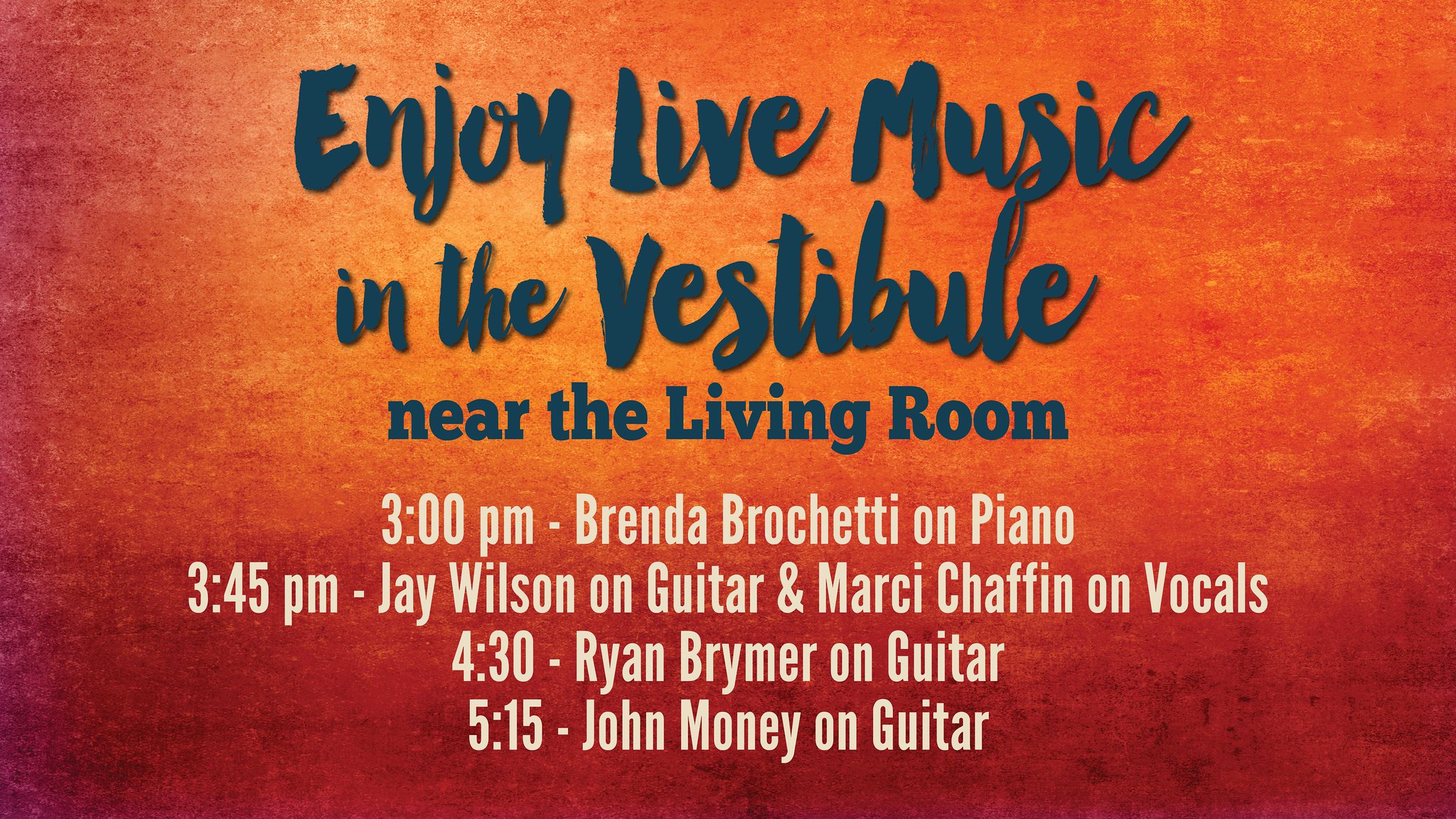The image is an advertisement with a burnt orange background transitioning to a lighter orange in the middle, enhancing the visibility of the text. The advertisement features blue and white lettering with varying font styles. At the top, in an artsy dark blue font, the text reads, "Enjoy live music in the vestibule near the living room." Below, in a straight, normal blue font, it provides the schedule: "3 p.m. Brenda Brochetti on piano, 3.45 p.m. Jay Wilson on guitar and Marcy Chaffin on vocals, 4.30 p.m. Ryan Bremer on guitar, 5.15 p.m. John Money on guitar." The event details at the bottom are in a simple white font against the orange background, clearly indicating the line-up of musicians and their respective performance times.